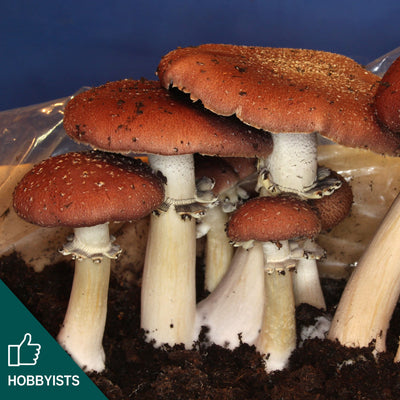This close-up, ground-level photograph showcases a cluster of seven mushrooms growing out of black dirt. Spanning a small, vertical rectangular frame, the mushrooms, with their curved creamy white stems and dark reddish-brown, dome-shaped caps adorned with light brown flecks, stand strikingly against a stormy blue background. The dirt appears to be contained with some type of plastic layering behind the mushrooms. In the bottom left corner of the image, a teal blue triangle features a white thumbs-up icon and the word "HOBBYISTS" in bold capital letters. The mushrooms, varying in size from small to large, intermingle, with larger ones predominantly standing tall and smaller ones nestled between them.